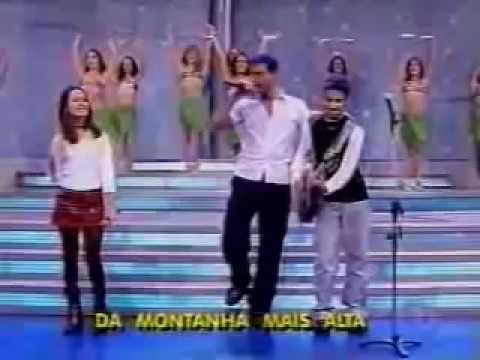In this image, a scene from a music television show is captured with vibrant detail. The stage features a lower flat area with a blue surface, and behind it, a flight of blue and purple stairs leads up to a larger platform. At the top of the stairs, a group of six female dancers, dressed in golden bra tops and blue and green skirts, all striking a pose with both arms raised high.

In the foreground, three individuals stand by the steps. On the left, a young woman with long, shoulder-length hair wears a white blouse, a very short red skirt, black leggings, and black shoes. She stands confidently beside two men. The man in the center has black hair and is dressed in a short-sleeved white button-up shirt, with the top buttons undone, black pants, and black shoes, holding a microphone. To his right, another man plays a black acoustic guitar with a white strap and wears a black shirt with white sleeves, gray pants, and brown shoes.

The image is framed by yellow text with black borders reading "Da montanha mais alta," and a microphone stand is visible in the bottom right corner, adding to the lively and dynamic ambiance of the performance.